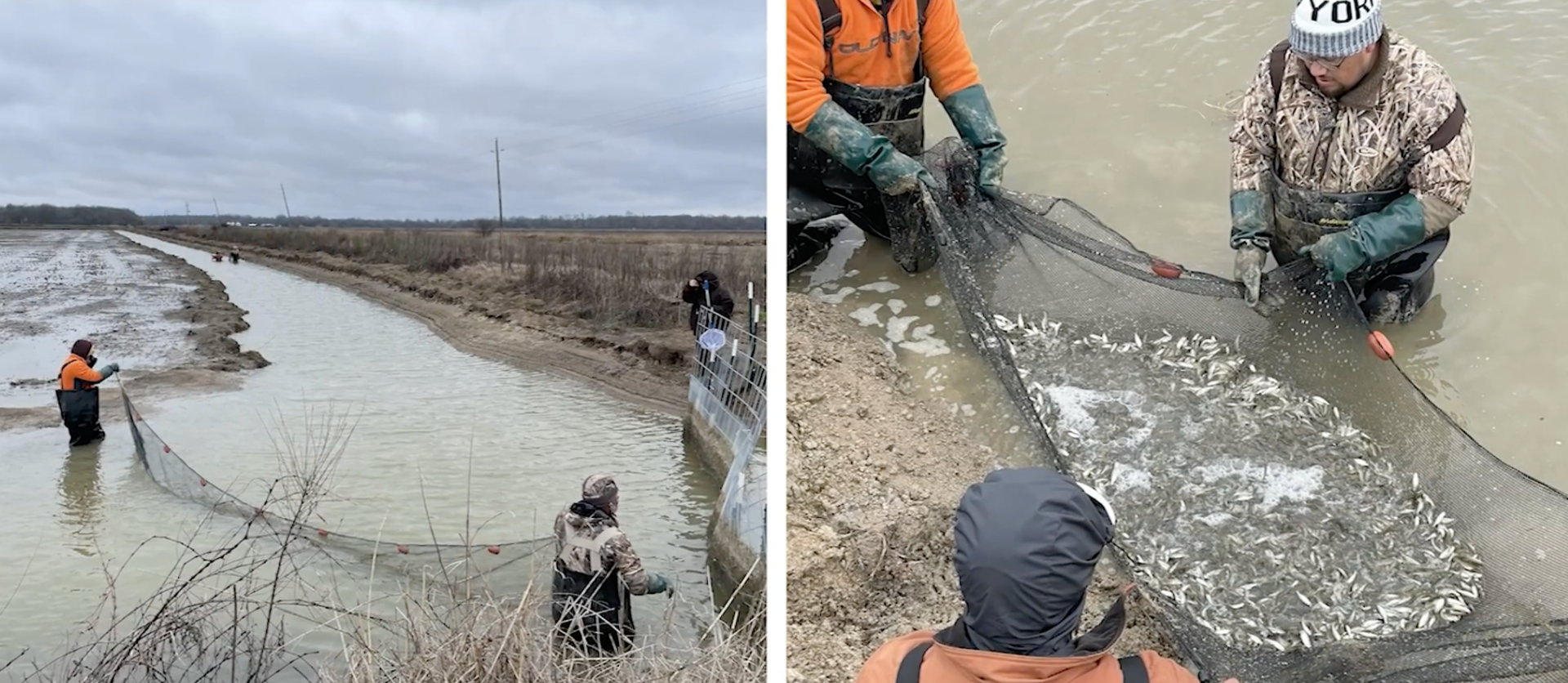The image consists of two side-by-side square photographs taken in the same location, likely by a body of murky water on a cloudy day. In both photographs, two men are wearing waders and are engaged in some form of aquatic activity, possibly scientific research or fish collection. In the left photo, the men are standing in a canal or ditch filled with water, each holding one end of a large black net. A third person stands on the bank watching them. In the right photo, the two men, now joined by a third person, have brought their nets together and are examining their catch. The net is filled with small silver or gray fish, and the men appear to be focused on the contents. One man wears a bright day-glow orange top, while another sports a pull-down knitted cap with the word "York" partially visible. The trio seems engaged and possibly pleased with their netted haul.